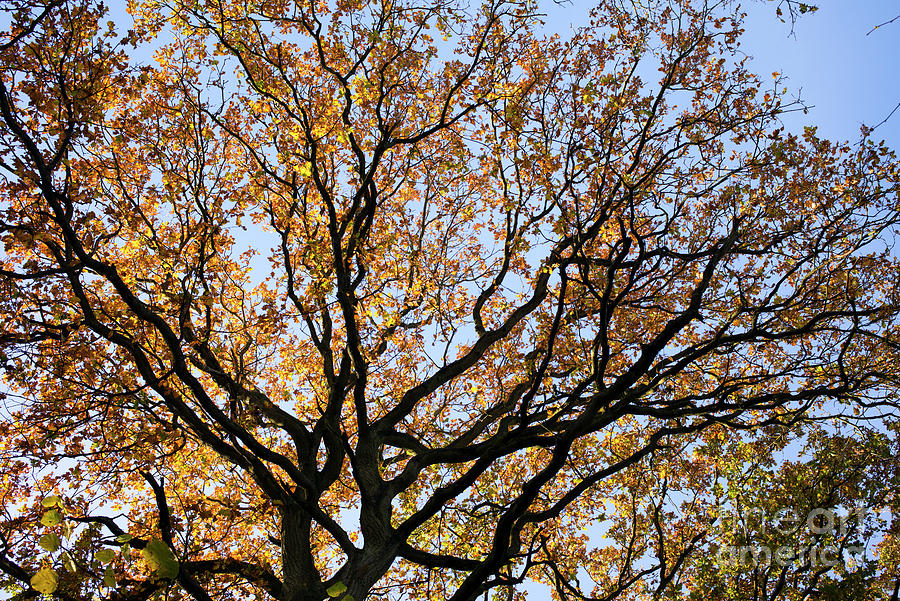This is a vibrant color photograph taken outdoors in autumn, showcasing the intricate beauty of a tree captured from a low angle. The tree, standing tall and central in the frame, has its many branches stretching upwards, adorned with leaves that display the rich fall colors of orange, yellow, and a hint of brown. The sunlight bathes the leaves, creating a play of shadows over the dark-toned, curving branches of varying thicknesses. The background reveals a clear blue sky, accentuating the seasonal hues of the foliage. In the lower right-hand corner of the image, a partially obscured watermark is visible, presumably reading "Heart America." This watermark is somewhat difficult to discern entirely due to the overlapping leaves. The lack of clouds in the sky and the crisp detail of the leaves and branches provide a serene and detailed capture of a quintessential autumn day.